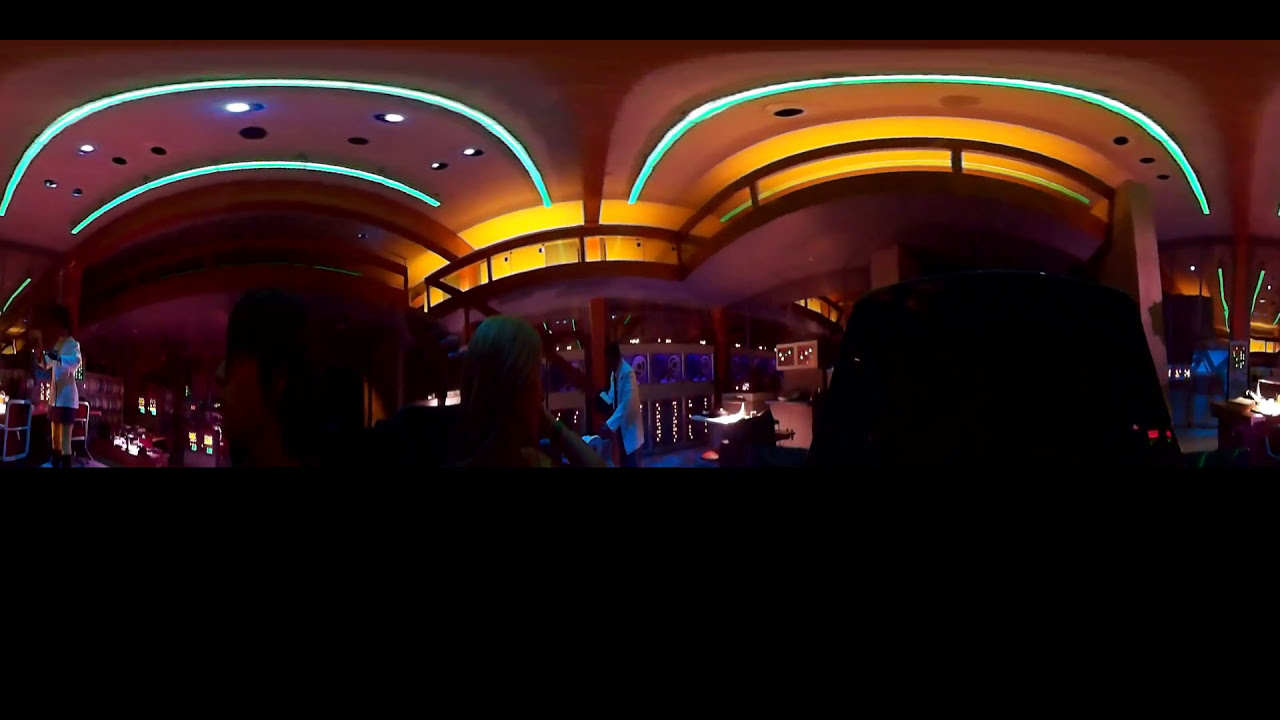The image depicts a dimly lit interior scene that exudes a futuristic and somewhat surreal ambiance, akin to a science fiction setting. The ceiling features wooden paneling with a yellow glowing light running through it, and a light green neon strip arches overhead. White spotlights intersperse the neon, contributing to the overall illumination. The walls are adorned with futuristic, white accent lights reminiscent of those seen in classic science fiction films, further enhancing the technological vibe. The background is predominantly dark, creating a stark contrast with the illuminated elements.

In the foreground, to the bottom left, stands a person in a white shirt and dark shorts, while centrally positioned is another individual dressed in a long white jacket or suit jacket. The image appears panoramic, with parts of the room stitched together in a warped, fisheye-like perspective, making the structures seem unusually positioned and giving a flat yet rounded appearance.

A stage is also visible, suggesting a performance space, potentially for singing. The stage is accentuated by purple and orange lights on the walls, adding to the vibrant yet mysterious atmosphere. A cluster of tables is set up within this space, contributing to the impression of a casino or bar. Overall, the image captures a highly detailed, almost otherworldly environment, blending elements of the familiar with the futuristic.